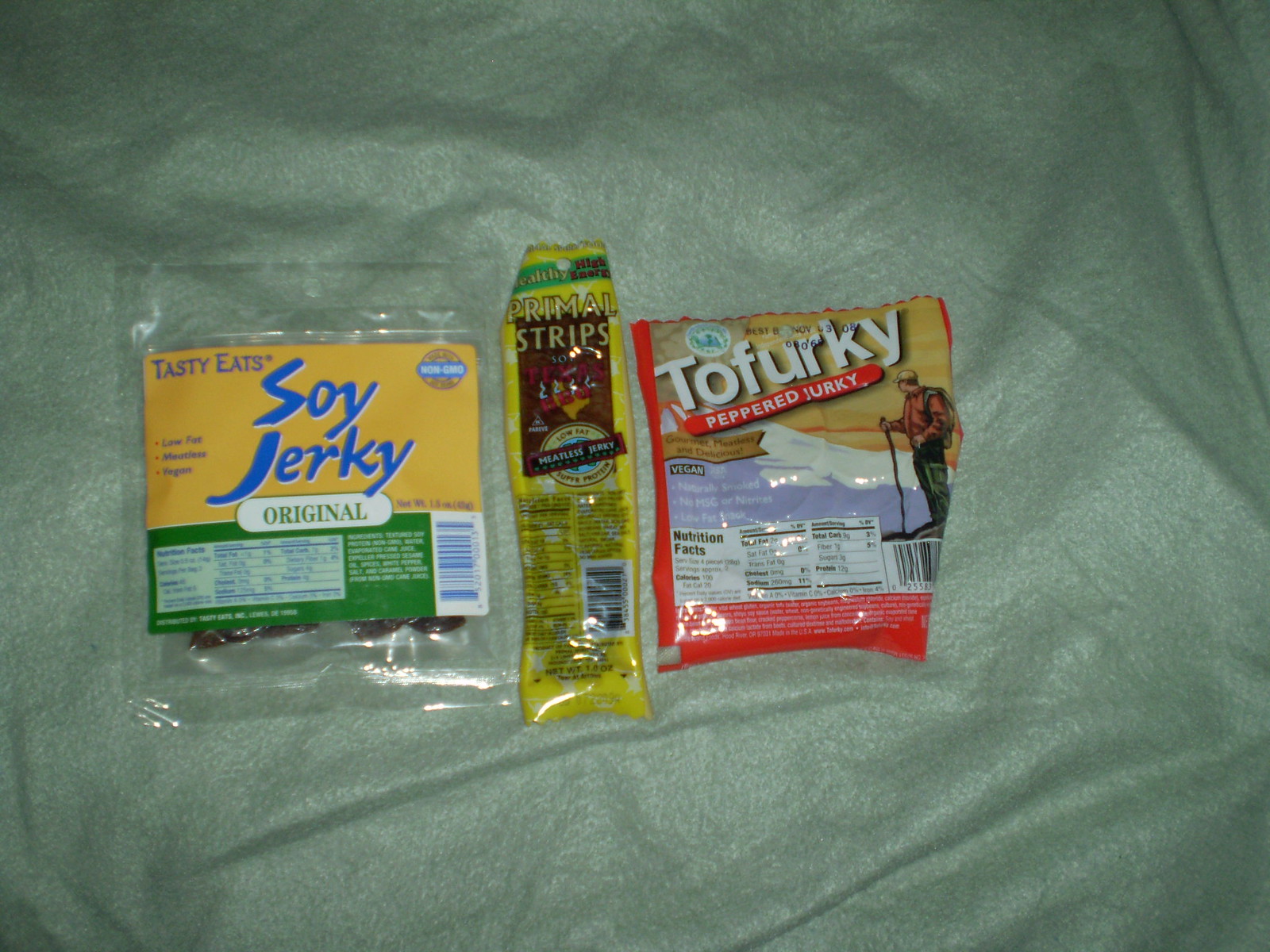The image shows three different packages of non-meat jerky products lying on a pale, grayish-green, shiny, wrinkled cloth. The package on the left is square and plastic with a yellow and green label. It displays "Tasty Eats" in black text, "soy jerky" in blue text, and "original" in green text over a white oval, along with product information on a green area. The middle package is rectangular and yellow, branded as "Primal Strips," which is a type of meatless jerky. The third package, on the right, is square and gold with a red trim, labeled "Tofurky" and "peppered jerky." The Tofurky package also features an image of a man skiing or hiking near a mountain and includes nutrition facts on the front.